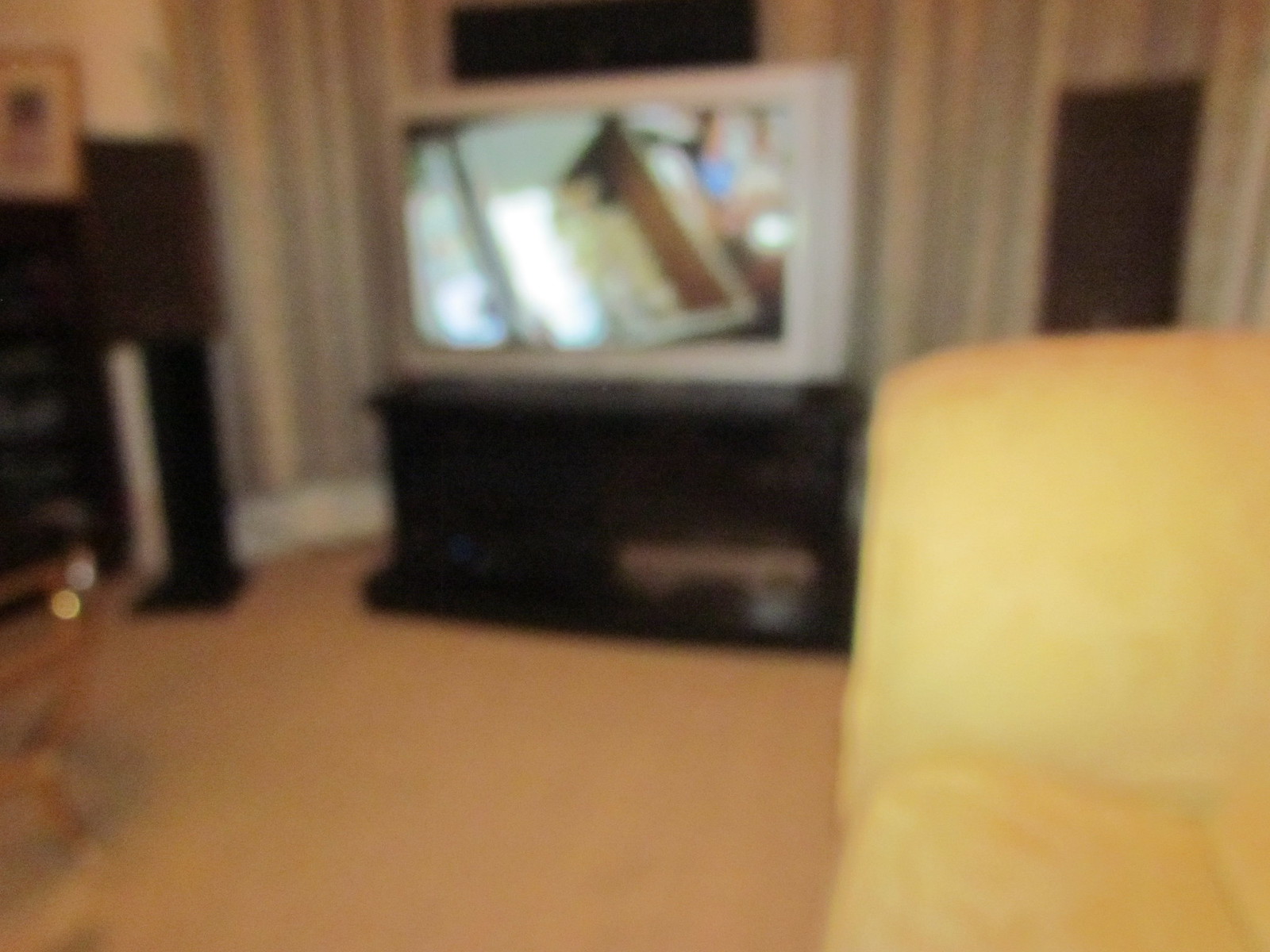This image appears to be a blurred, indoor color photograph taken in what seems to be a living room. The room features a light-colored carpet, potentially beige or orangish-brown, extending across the floor. The walls in the background are adorned with a wallpaper featuring vertical gray and white stripes, complemented by white floor molding trim along the bottom. Central to the photograph is a black or dark brown low TV stand, upon which sits a large, potentially retro TV with a silver outline. The TV is on, displaying an indistinct image. To the left of the TV stand, there is a large piece of brown or black furniture, perhaps a credenza, with a framed picture on it. Additionally, a vertical black stand with a rectangular black speaker is seen to the left of the TV. In the upper right corner, a yellowish object, likely the edge of a sofa, is partially visible, along with another brown speaker. No text or print is visible in this photograph.